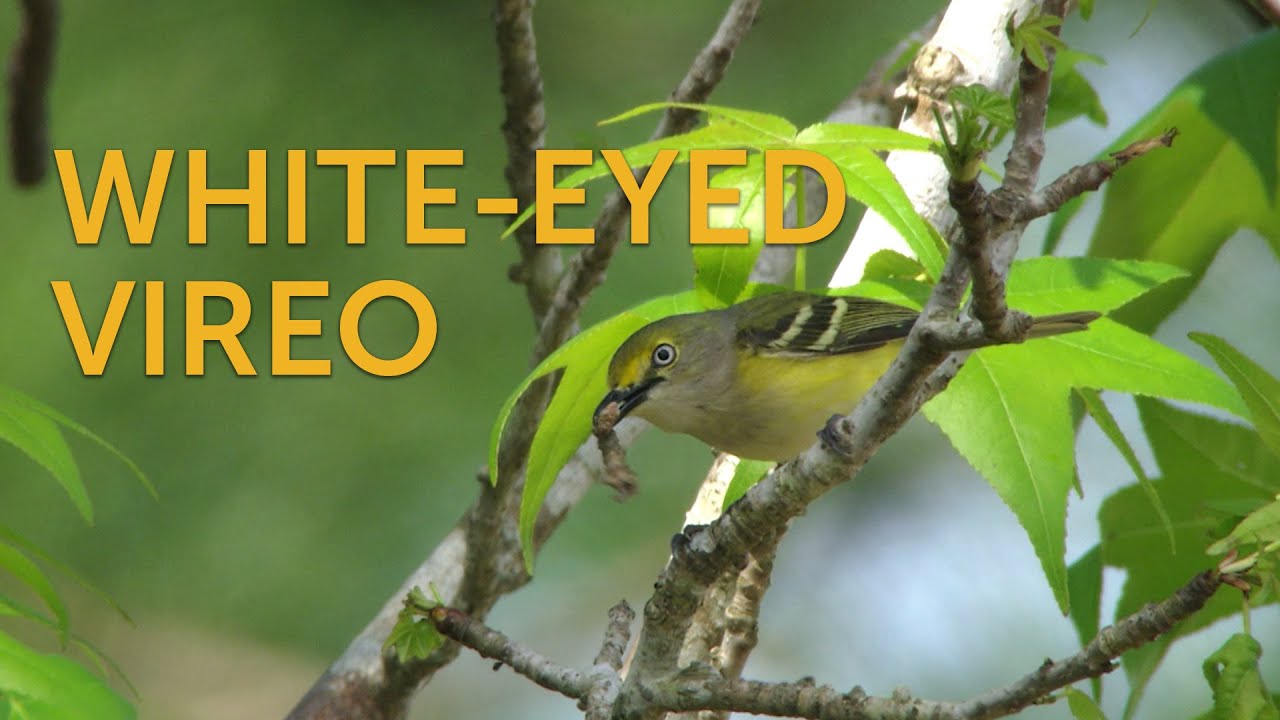This vibrant and detailed image features a close-up of a White-Eyed Vireo perched on a branch amidst newly sprouted green leaves, suggesting a springtime setting. The bird boasts a striking appearance with a yellow belly, yellow tinges around its eyes, and a darker brown plumage accented by black, white, and possibly gray stripes across its wings. Its beak, which appears to be holding something indistinct, is black, and it has characteristic black eyes. The background is artistically blurred, drawing focus to the bird. The accompanying large, black, orange-tinted text spells out "White-Eyed Vireo," making this photo, with its nature-rich composition and clear subject focus, suitable as a thumbnail for a YouTube video or the header image of a website. The image thus offers a glimpse into nature, capturing the bird seemingly gazing back at the viewer, creating an engaging and serene visual experience.